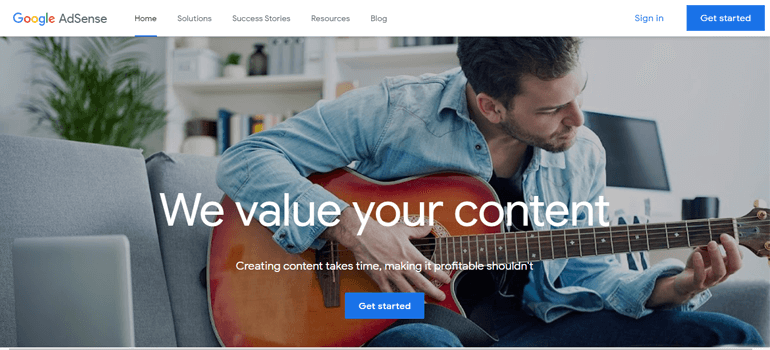The image is an advertisement for Google AdSense. In the upper left corner, the Google logo is prominently displayed, accompanied by the "AdSense" branding. There are five clickable sections in the navigation menu, with the "Home" section highlighted. On the right side of the top bar, there is a clickable blue "Sign In" text, and next to it, a blue button with white text that reads "Get Started."

The central piece of the ad features a visual below this header. It depicts a man in his late 20s, seated on a white couch, actively playing a guitar. He has brown hair and is dressed in a long-sleeved denim shirt. His right hand is positioned on the bottom half of the guitar while his left hand strums the strings. The room's background includes a plant, adding a touch of greenery to the setting. This scene likely aims to evoke a sense of creativity and relaxation, aligning with the ad’s intention to promote AdSense as a tool for creators and entrepreneurs.